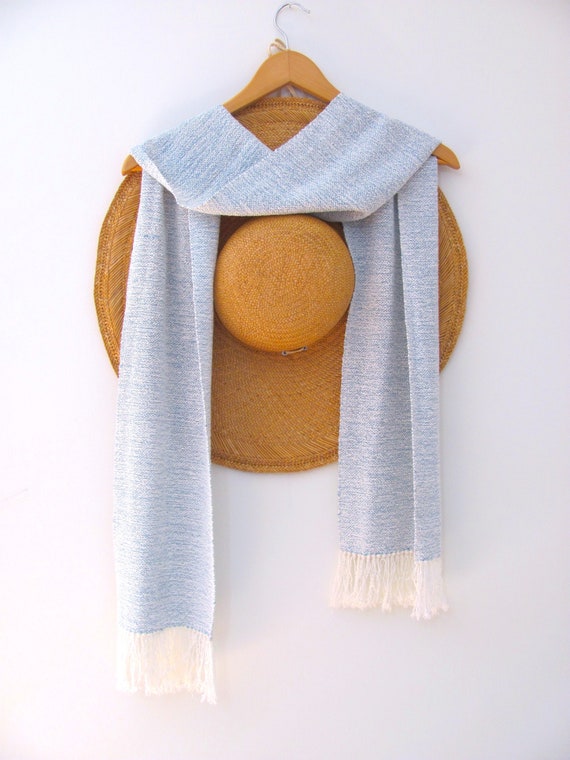This photograph features a wooden clothes hanger suspended from a nail on a very light gray wall. Draped over the hanger is a light pastel blue scarf with white fringes dangling from each end. The scarf is neatly arranged in a V-shaped formation, with one side hanging slightly lower than the other. Nestled behind the scarf and also hanging from the same nail is a wide-brimmed, natural brown straw hat. The hat's generous brim extends beyond the edges of the scarf, providing an additional layer of texture and color to the composition. The metal hook of the hanger is visible, securing the arrangement on the wall. The clean, light-colored background ensures no distractions, keeping the focus on the intricately detailed hat and scarf combination.